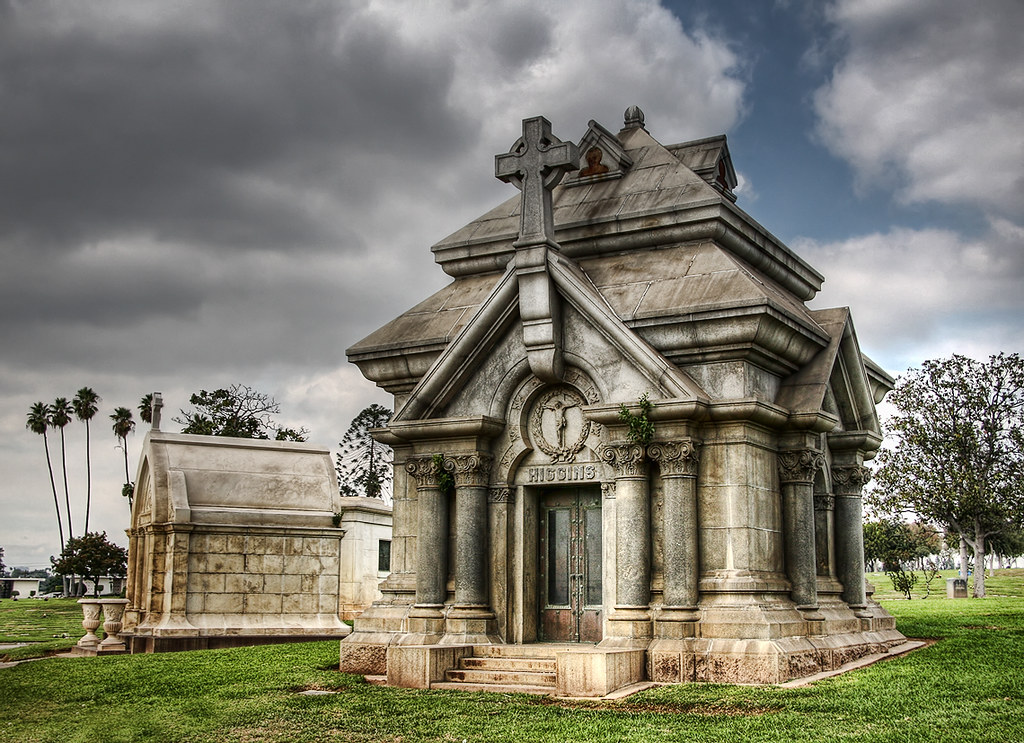In the image, there are two adjacent mausoleums situated in a cemetery, surrounded by green grass and set against a cloudy sky with patches of blue visible. The primary mausoleum, placed almost centrally, is composed of stone and has a distinct, church-like appearance. It features several round pillars on its exterior and has a series of steps leading up to its stone double doors, which are secured with metal latches. The structure is topped with a large cross, and just above the doors, there is a circular depiction of Jesus on the cross, accompanied by the name "Higgins." The roof is designed with a double-layered effect, and there are windows on the upper section of the roof, one of which contains stained glass illustrating a head and shoulders. 

To the left of the main mausoleum lies a smaller, equally worn and old mausoleum, also made of stone, with white stone vases in front of it, one of which has foliage growing from it. The background showcases various trees, including palm trees. Additionally, on the right-hand side of the image, nearby one of the trees, there appears to be an indeterminate stone or box-like structure. The overall setting conveys a somber and historic atmosphere, emphasized by the weathered condition of the mausoleums and the overcast sky.